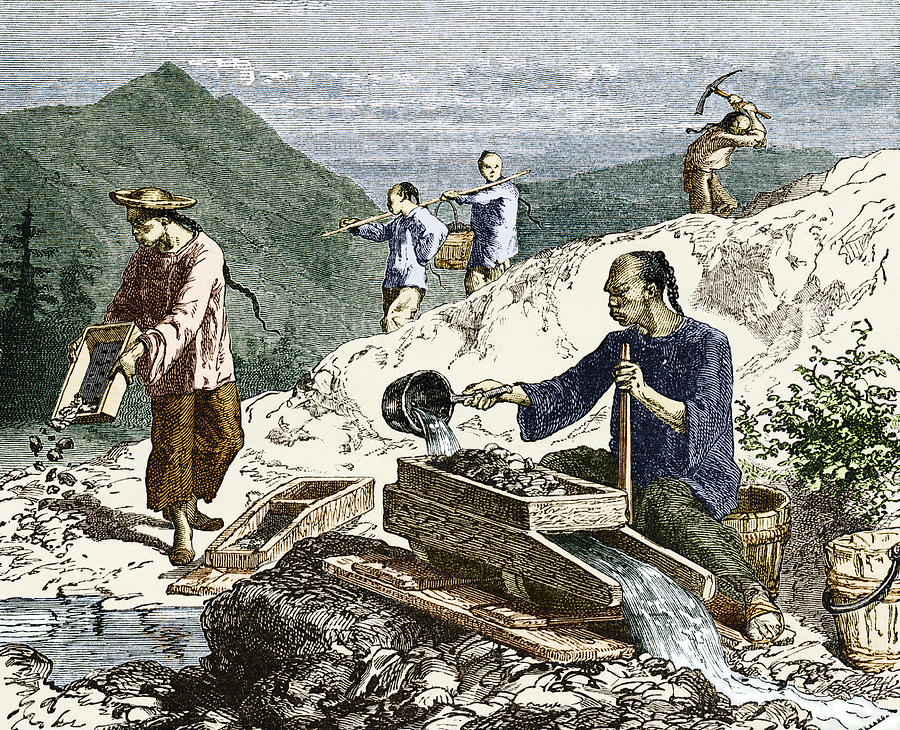This illustration, reminiscent of a woodcut or inked comic style, depicts what appears to be Chinese laborers during the California Gold Rush. The foreground features a central figure sitting on a wooden bucket, dressed in a dark blue tunic and forest green pants. This man, with traditional long ponytail and slightly exaggerated facial features, is seen pouring water through a sluice box atop a dammed stream, which is used to sift through mined rocks for gold.

To the left, another worker wearing a red, flat-brimmed straw hat, a long-sleeved pink shirt, brown pants, and sandals, is seen emptying a rectangular gold-sifting pan into the stream. Adjacent to him is a small sluice box, partially submerged in the water at his feet.

In the background, green hills and faintly detailed clouds serve as a scenic backdrop. On the upper right, a laborer is captured mid-action with a pickaxe against a beige hill. He is dressed in a brownish shirt and pants, sans hat, revealing his long ponytail contrasting with his shaved forehead.

Further to the middle right, two additional workers, also with traditional long ponytails, are seen transporting a bucket suspended from a pole shared between their shoulders. They are dressed in blue tunics and whitish brown pants, walking one in front of the other along the hillside.

The entire scene is marked by minute details, from the flowing water through the sluice box to the fine lines depicting the workers' attire and the surrounding foliage, vividly illustrating the labor-intensive process of gold mining.